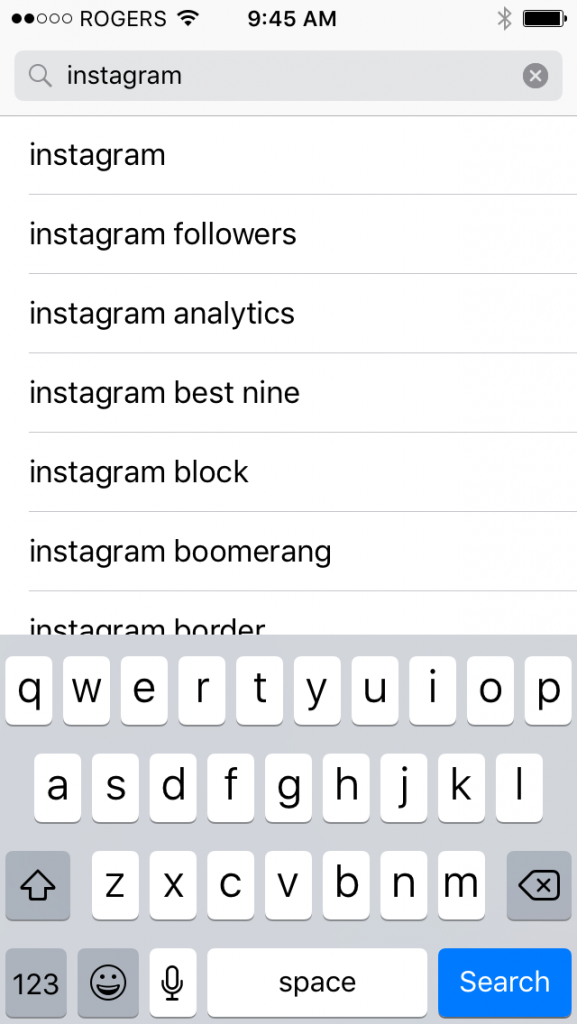This mobile screenshot captures a detailed view of a smartphone display. The top portion of the image is predominantly white, creating a clean background. Prominently displayed at the upper left-hand corner, in bold black capital letters, is the word "ROGERS." To the left of this word are two filled circles followed by three empty ones. Adjacent to these is a WiFi signal icon. Centered at the very top of the screen is the current time, reading 9:45 AM. On the upper right corner, icons for Bluetooth and battery status are neatly lined up.

Just below the top white section lies a horizontal gray search bar featuring a magnifying glass icon on its left end. Inside the search bar, the user has typed "Instagram," and on the right end of the bar, a circled 'X' icon is present, allowing for the clearing of the search term.

Below the search bar are search results, which are separated by thin gray horizontal lines. The list includes: Instagram, Instagram followers, Instagram analytics, Instagram best 9, Instagram block, Instagram boomerang. The final entry, partially obscured by the keyboard, reads "Instagram border."

The lower portion of the image, dominating the bottom area, is a virtual keyboard with a light gray background and black letters. This keyboard layout comprises three rows of alphabetic characters. Key functional buttons are arrayed around these rows: an up arrow, a left arrow, a "123" button, an emoji button, a microphone button, and a spacebar. Positioned at the bottom-right corner in a blue button is the word "Search" in white font.